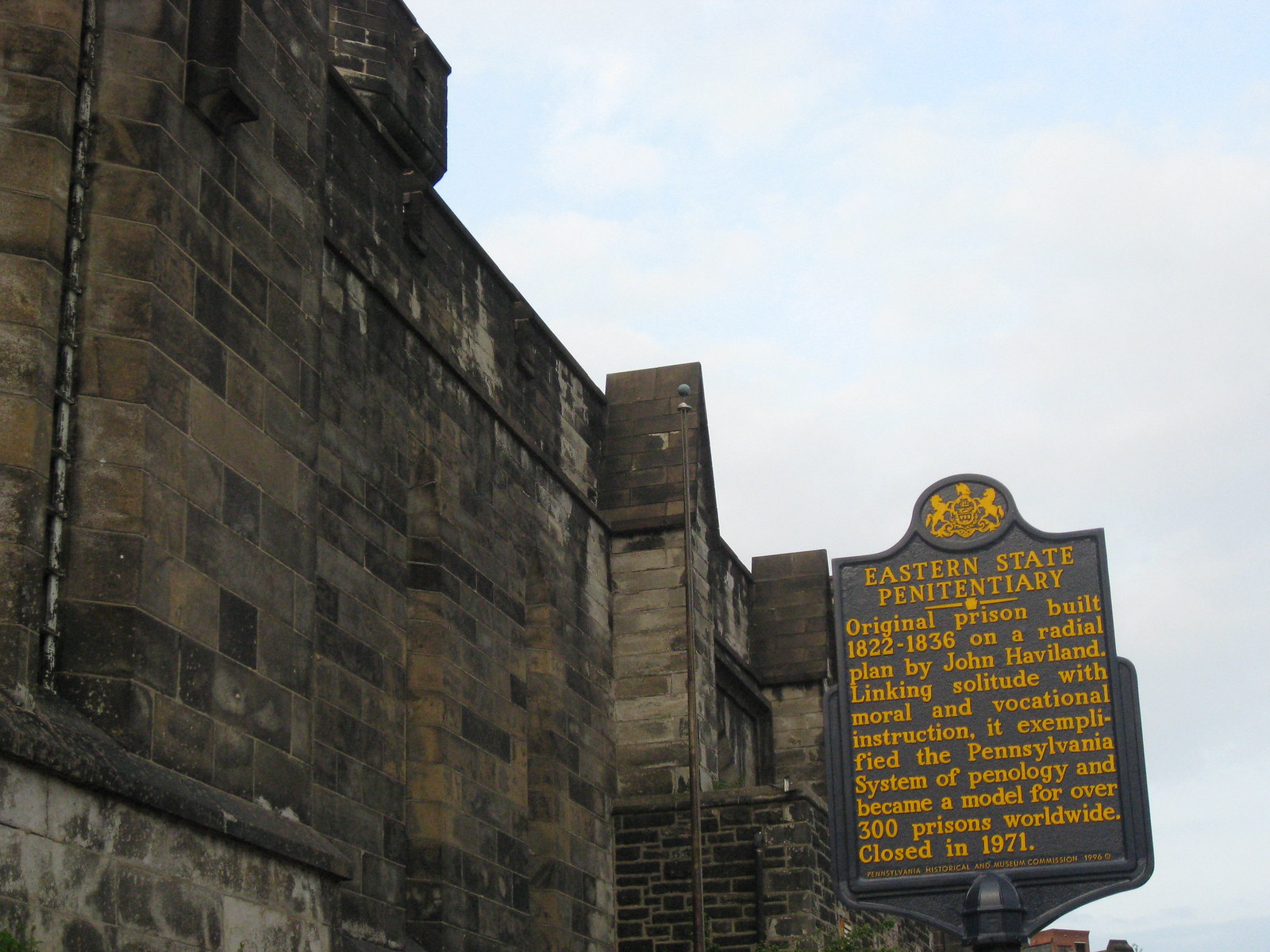This photograph captures a weathered, medieval-looking gray stone prison wall of the Eastern State Penitentiary, showcasing the bleak and grim atmosphere with dark grays, tans, and weather-stains of browns, grays, and blacks. The wall's thick cinder blocks stretch upward towards a cloudy blue sky that occupies the top-right portion of the image, adding contrast to the scene. In the bottom-right corner, a prominently mounted metal sign with a circular emblem atop – featuring a gold shield flanked by horses and a plume – sticks out from the wall. The bold goldenrod text on the sign reads: "Eastern State Penitentiary, original prison built 1822-1836 on a radial plan by John Haviland. Linking solitude with moral and vocational instruction, it exemplified the Pennsylvania system of penology and became a model for over 300 prisons worldwide, closed in 1971." The entire composition suggests an outdoor shot captured during daytime, with a slightly wider-than-tall view, slanting downwards to the right.